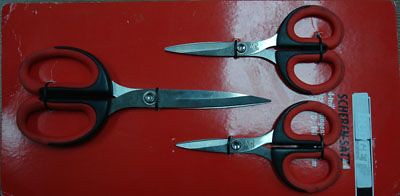This horizontal photo features three pairs of scissors displayed on a red background. The largest pair of scissors is positioned centrally, pointing to the right, with black handles accented by red on the inner circles and a silver metal blade. Flanking this larger pair on either side, pointing left, are two smaller scissors of identical size and design, with red handles encircled in black and silver blades. Beneath the two small scissors, on the right side of the photo, is a patch of white that could be powder, paint, or crayon. A black line, resembling a tie or packaging strap, runs over the scissors, adding to the impression that they are part of a set. There is also a faint text on the red background, possibly reading "sheer sat," along with some white markings above it, which are hard to read. A tube-like object lies to the right of the smaller scissors, its purpose or content unclear.